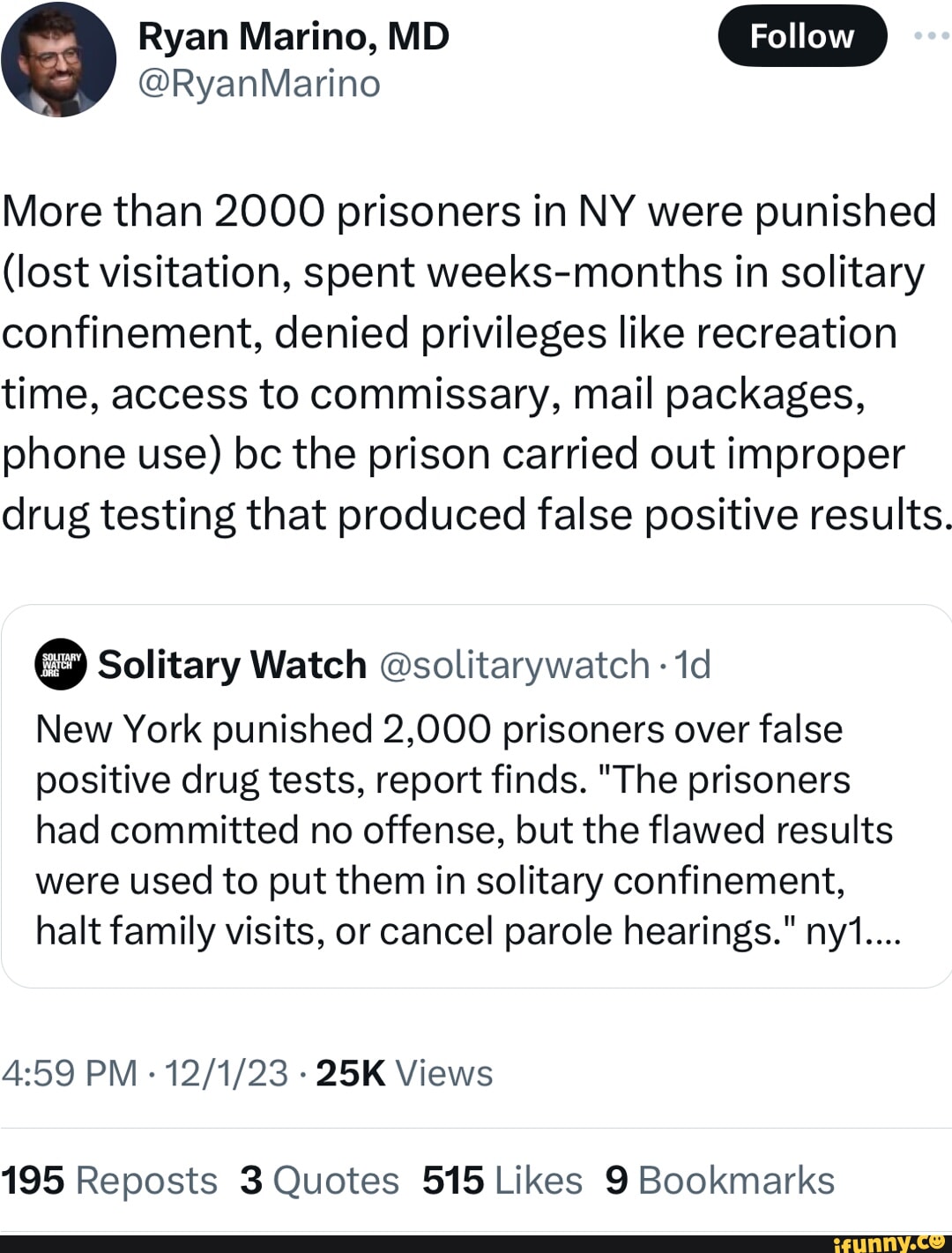This is an image of a tweet featuring a post by Ryan Marino, MD. The background is predominantly white, except for a thin black border at the bottom right corner, where "ifunny.c" is written in yellow with a smiley face. In the top left corner of the tweet, there's a profile picture of a man with brown hair, a beard, and glasses, against a black or dark blue backdrop. 

To the right of the profile picture is Ryan Marino's name in bold black letters, followed by a black "Follow" button and an ellipsis. Below his name, in gray text, appears his handle, @RyanMarino. The tweet consists of six lines where Ryan Marino discusses the punitive measures against prisoners in New York, mentioning issues like solitary confinement and revoked privileges.

Further down, there is a reply indicated by a small square with a black circle and white lettering for the profile picture, identified as "Solitary Watch" in bold letters and @solitarywatch in gray, marked as one day old. The reply consists of five lines detailing the punishment of around 2,000 prisoners due to false drug tests and subsequent reports.

At the bottom left of the tweet, the timestamp reads 4:59 p.m. · 12/1/23, followed by "25k views" in bold. Next to it are interaction counts in gray and bold: 195 reposts, 3 quotes, 5,015 likes, and 9 bookmarks.